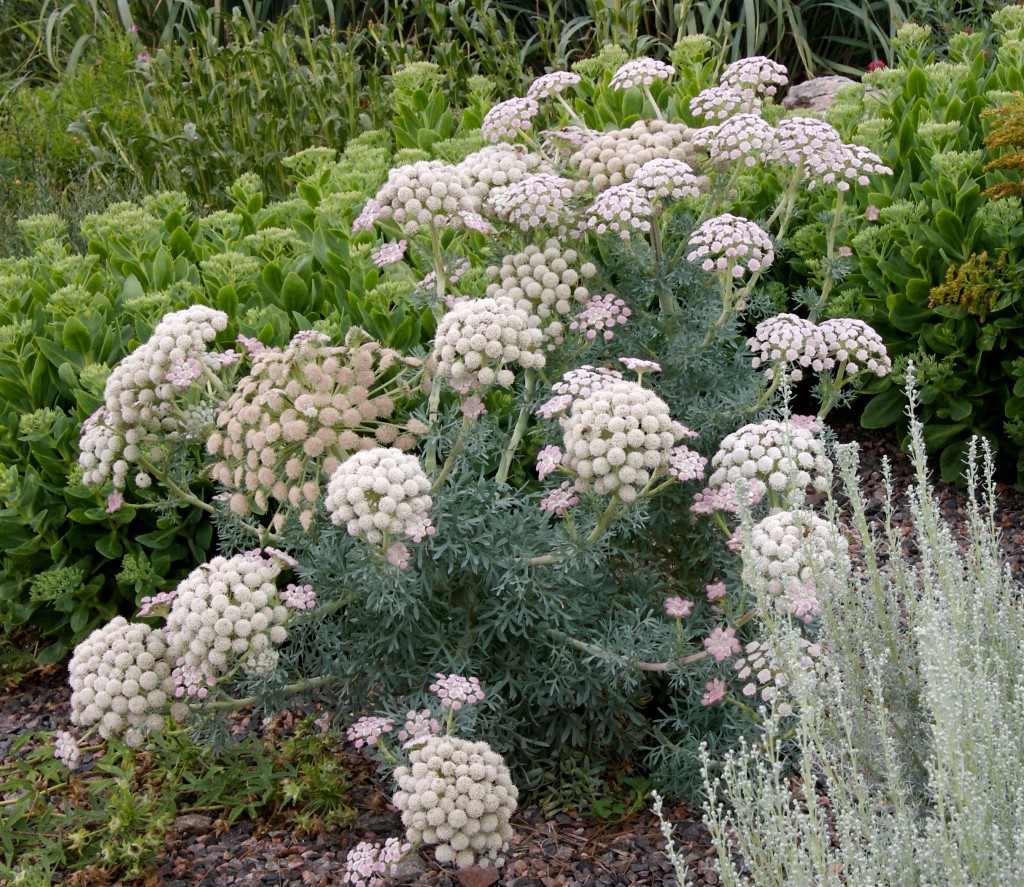In this detailed outdoor image, a mixed array of wildflowers and dense vegetation are showcased, suggesting a natural forest or wilderness setting rather than a garden. Dominating the foreground is a lush, fern-like flowering shrub with numerous white, lace-like flowers that form full, dome-shaped clusters, resembling cotton balls. Intermingled among these are green stems and foliage, some of which have yet to bloom. On the lower right, you can spot smaller white bushes with slender stems ending in tiny white balls. The colors mainly comprise green and white, highlighted by occasional hints of pink buds peeking through the foliage. The background transitions into wild grasses and overgrowth, punctuated by a variety of green plants, contributing to the sense of an untamed, open field. Scattered across the ground in the lower left and middle are various small, colorful rocks, adding texture to the natural scene.